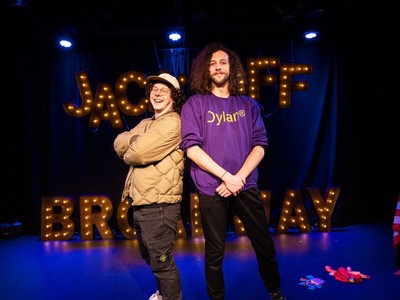This detailed photograph captures two Caucasian male performers standing on a stage, partially obscuring a large lit-up marquee behind them. The marquee features bold black letters illuminated with multiple light bulbs, with the visible sections spelling out "J-A" at the beginning and "F-F" at the end, suggesting it might read "Jack off Broadway." Below, "Broadway" is clearly spelled out along the ground level. The stage itself is dimly lit, with three distinct lights and a black curtain background accentuated by red and blue splotches.

The shorter man on the left wears a baseball cap, glasses, a tan jacket, tan pants, and white shoes. He has short curly hair and is positioned with his back to the taller man. The other man is taller and sports long, wavy hair, a mustache, and beard growth. He dons a purple sweatshirt with the word "Dylan" printed on it, with the sleeves rolled up to his elbows, and black pants. He is posed holding his wrist, adding a casual yet dynamic element to their stance.